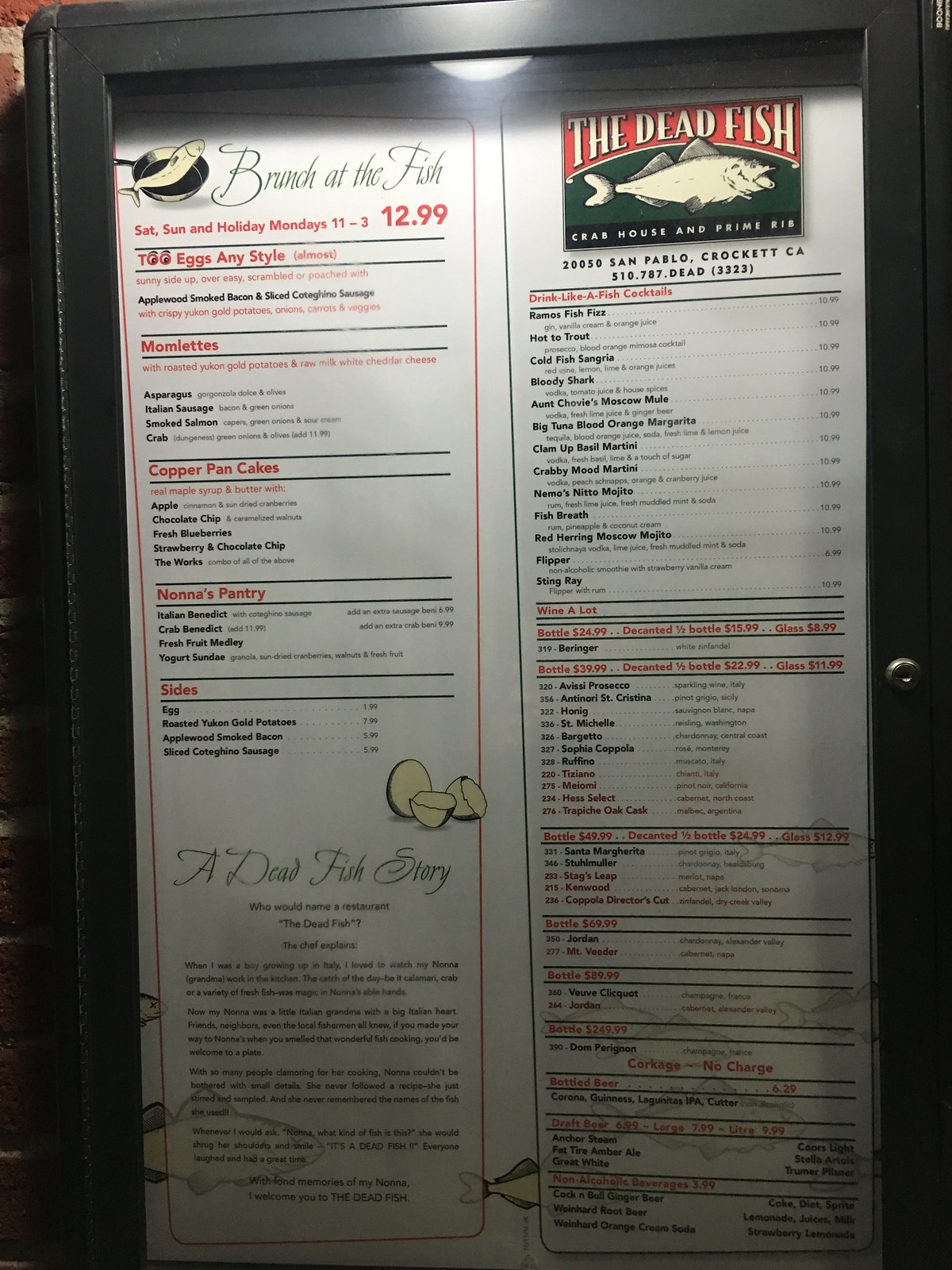A photograph captures the menu display of The Dead Fish restaurant, encased behind a reflective glass pane in a black metal frame. The menu box, securely locked with a silver lock, is affixed to a section of the brick exterior of the building. Positioned at the top, a light illuminates the menu, ensuring its contents are easily readable. The display boasts the restaurant’s distinctive logo: a vibrant red graphic with white lettering, featuring a green lower section adorned with a white fish detailed with gray scales. Below the logo, a black banner bears the text "Crab House and Prime Rib." The focal point of the menu highlights "Brunch at the Fish," available Saturdays, Sundays, and holiday Mondays from 11:00 AM to 3:00 PM for $12.99, and lists an array of breakfast and fish options. At the bottom, a section titled "A Dead Fish Story" invites readers to delve into the unique narrative behind the restaurant.